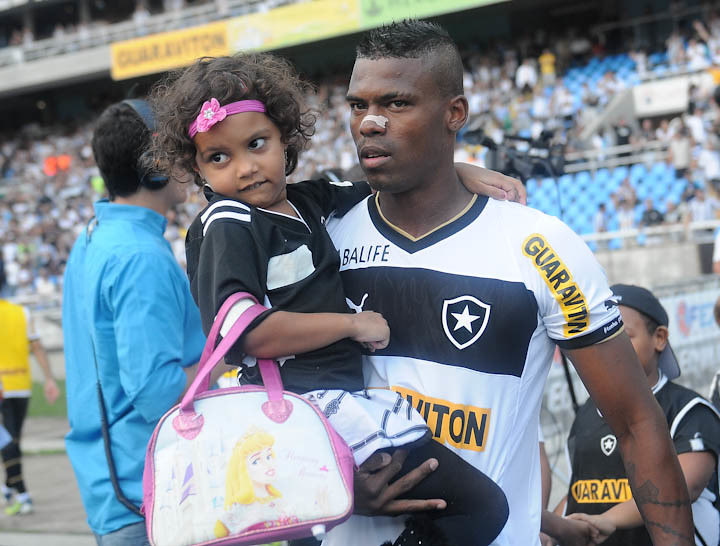In an image set in the bustling ambiance of a sports stadium, presumably post-match, a close-up captures a soccer player, distinguishable by his white jersey featuring a black banner across the chest with a shield emblem showcasing a star. The garment has a navy-bordered collar with gold accents. The player, donning a nasal strip and a very short cropped haircut, is seen holding his young daughter. The little girl, perhaps 5 or 6 years old, wears black pants and a black jersey-like shirt adorned with white stripes. A pink headband with a flower sits on her short bob haircut. In her hands, she clutches a white purse with pink borders and handles, possibly embellished with a Disney character. The background reveals the lower sections of a stadium, populated with blurred figures of spectators and banners of various sponsors, underlining the lively atmosphere of a sports event.